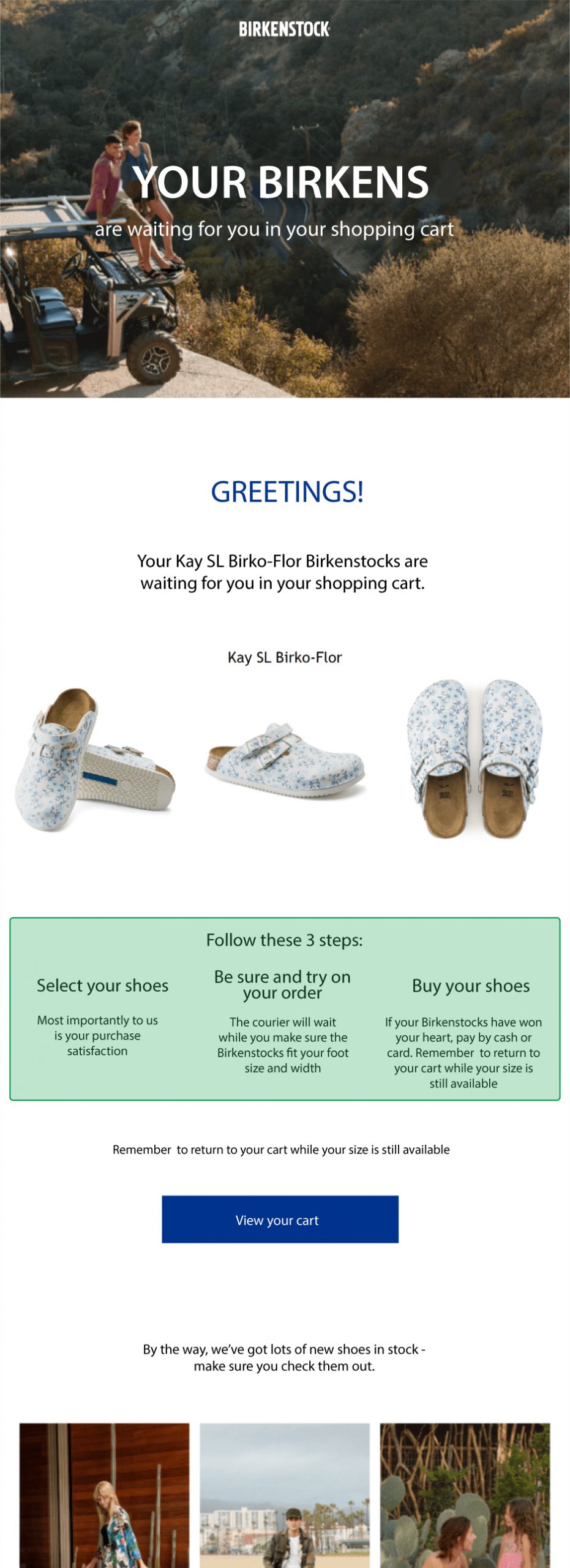This still image captures a detailed view of a Birkenstock website. At the top, a wide rectangular banner features a couple, a man and a woman, adventuring in the wilderness on an ATV. The background is vibrant with thick underbrush and towering mountains. Superimposed on this image in white text is the word "Birkenstock," along with an inviting message: "Your Birkens are waiting for you in your shopping cart." Below that, a friendly greeting stands out in blue text: "Greetings!"

The next section provides specific details regarding a pair of KSL Birko-Floor Birkenstocks, eagerly waiting in the user's shopping cart. The text reads: "Your KSL Birko-Floor Birkenstocks are waiting for you in your shopping cart," with the product name, "KSL Birko-Floor," prominently displayed in the center.

A series of images showcase the Birkenstocks from various angles for a comprehensive view: the first image on the left highlights the front toe and sole, the next shows a side view of the right shoe, and the final image provides a top-down perspective of both shoes.

Beneath this display is a mint green rectangle adorned with dark green text that guides the customer through the purchasing process. At the top center, it says, "Follow these three steps..." On the left, it starts with "Select your shoes." 

There are clear steps ensuring customer satisfaction: first, "Be sure and try on your order," with a note that the courier will wait while ensuring the Birkenstocks fit correctly. To the right, it recommends purchasing if the shoes win your heart, mentioning, "Pay by cash or card." It emphasizes acting quickly to avoid missing out: "Remember to return to your cart while your size is still available."

Center-aligned in black text is a reminder, "Remember to return to your cart while your size is still available." Below that, a blue rectangle with white text invites the user to "View your cart."

Finally, in black text centered at the bottom, it encourages exploring additional products: "By the way, we've got lots of new shoes in stock. Make sure you check them out." Three photos underneath illustrate various people in different settings proudly wearing their Birkenstocks.